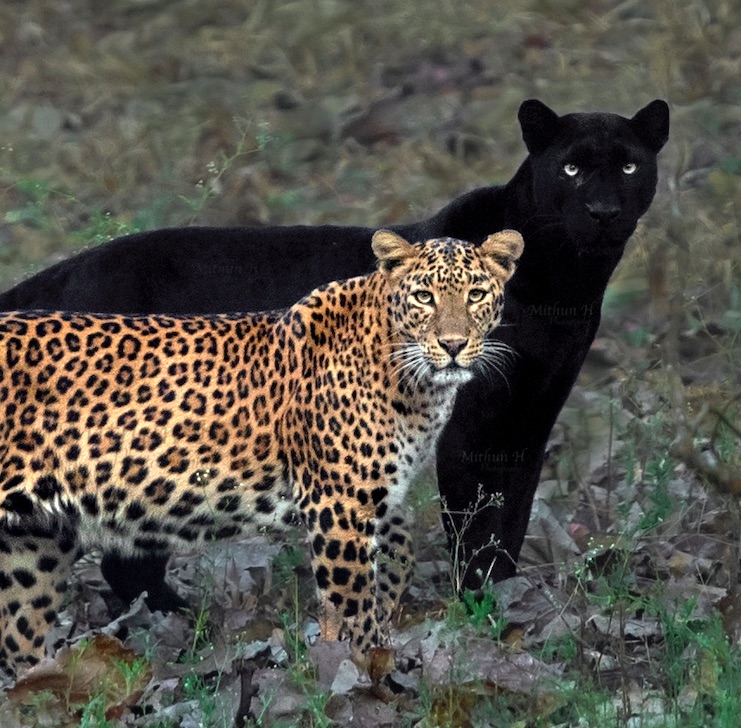The image portrays a pair of wildcats, a cheetah in the foreground and a black panther in the background, poised in a forest-like setting. The scene is overlaid with a thin layer of dead leaves, interspersed with patches of grass and a few rocky areas. Both felines have an intense gaze directed at the camera. 

The cheetah, closest to the viewer, features the characteristic black spots on its yellowish-brown fur, a white underbelly, thick white whiskers, and bright yellow eyes. Its body extends towards the left edge of the frame, with its front legs visible against the leaf-covered ground. Meanwhile, the black panther, standing a bit further back, is entirely black with striking yellow eyes and is partially obscured by the surrounding leaves and perhaps the cheetah itself. 

In the background, the scene blurs into what appears to be a mix of dirt, weeds, and grass, under a sunlit but seemingly overcast sky. A faint, nearly indecipherable watermark, "Mithen H," is also noticeable, primarily over the panther. Despite the differences in species, the two majestic cats share a captivating, almost fierce presence in the photograph.